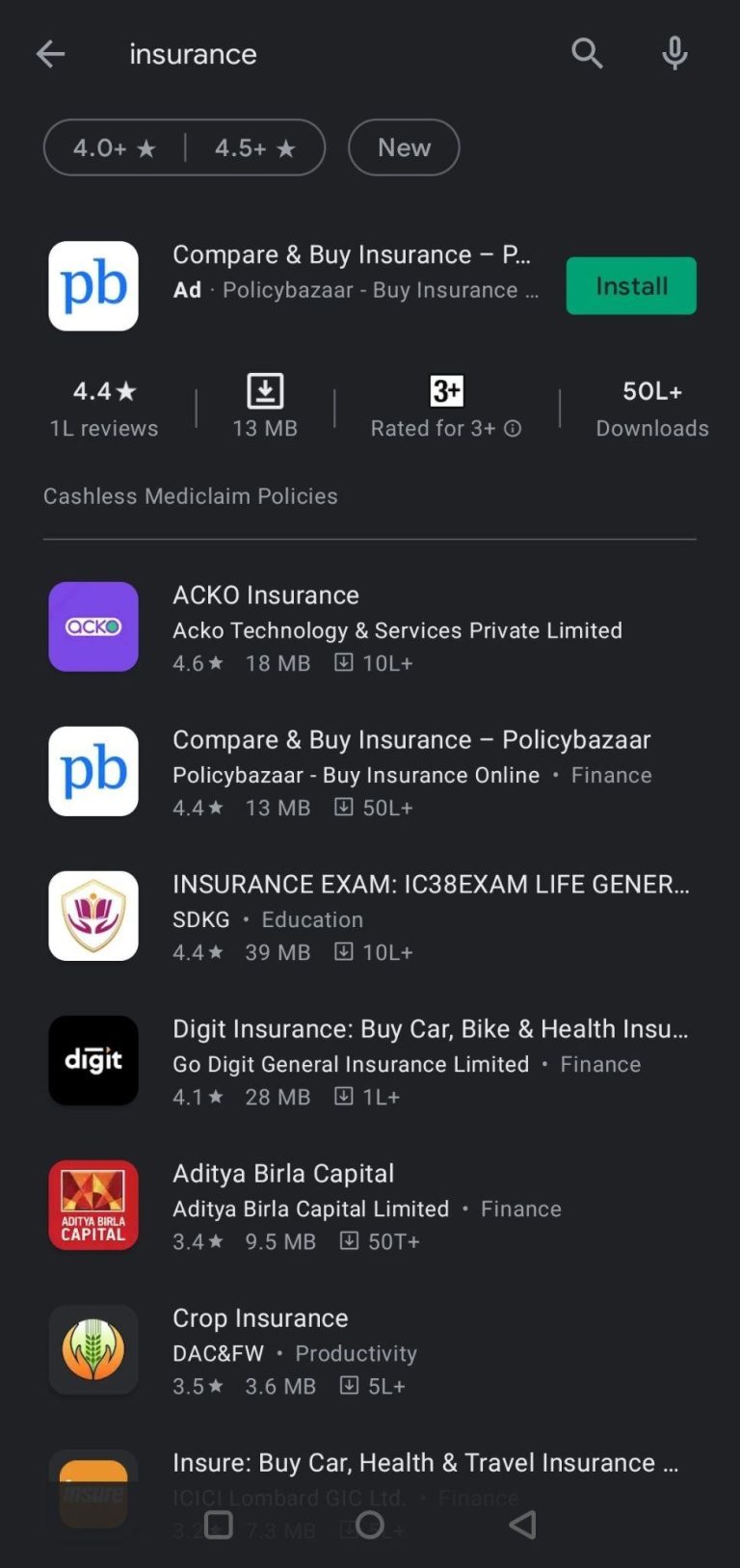This is a detailed caption of a screenshot from the Google Play Store showing search results for the term "insurance":

---

The screenshot depicts the Google Play Store search results for the query "insurance." In the upper left corner, there is a left-facing arrow, symbolizing a back button, adjacent to the word "insurance" in the search field. On the upper right corner, a microphone icon is present.

Just below the search bar, filters display options such as "4.0+ stars," "4.5+ stars," and a "New" button to refine the search results. 

The first app result is "PB company" with the tagline "Compare and Buy Insurance" and "Policy Bazaar." The app has a green "Install" button next to it. It is rated 4.4 stars based on 1L reviews, occupies 13 megabytes of space, is rated for ages 3 and up, and has over 5 million downloads.

Next in the list is "ACKO Insurance" by ACKO Technology & Services Private Limited. This app boasts a 4.6-star rating, is 18 megabytes in size, with 10 million-plus downloads.

Following that is an app named "Policy Bazaar" with the description "Compare and Buy Insurance, Insurance Quotes, Finance." It has a 4.4-star rating, weighs 13 megabytes, and shows over 50 million downloads.

Beneath these, additional app listings include "Insurance Exam," "Digit Insurance," "AD Trip by Large Capital," and "Crop Insurance," each providing various services related to insurance coverage and policy management.

---